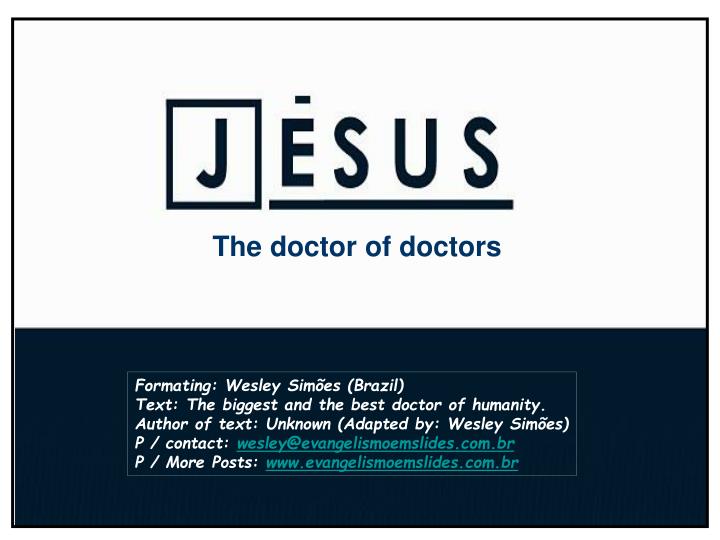The image is a large, square website post divided into two main sections. The top portion, occupying a bit more than half of the space, features a white background with the name "JESUS" in black, capitalized letters. The "J" is enclosed in a black frame, and the rest of the letters, "E-S-U-S," are underlined by a thick black line. Below this, in dark blue print, it reads "The Doctor of Doctors" in a mix of upper and lower case letters.

The bottom portion has a dark blue background with white text, displaying various details in a structured format. It starts with "Formatting, Wesley Simoes (Brazil)" followed by "Text, the biggest and the best doctor of humanity." The line "Author of the text: unknown (Adapted by: Wesley Simoes)" follows. Below this, a contact email is provided: "Wesley at Evangelistsamoasslides.com.br." The final line directs users to more content with "For more posts: www.evangelistsamoasslides.com.br". 

In summary, the poster highlights Jesus as "The Doctor of Doctors" and features formatted text adapted by Wesley Simoes, with additional contact information and a link for further posts.